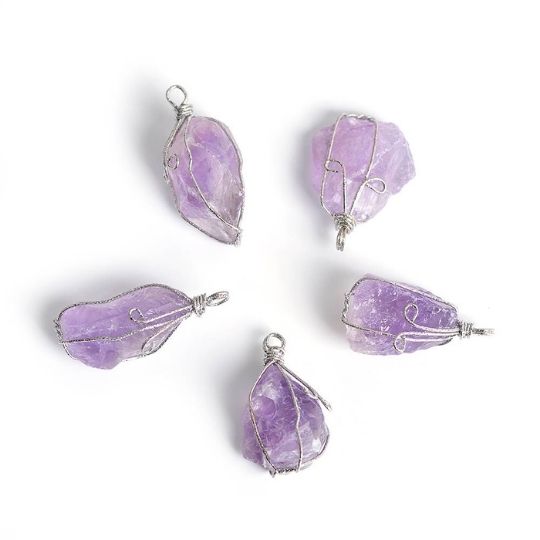This image captures five pale purple, rough, and uncut gems, believed to be amethysts, carefully encased in intricate silver wire settings. Each gem, approximately the size of a thumbnail, is artistically framed with polished and reflective thin wires that form loops at the top, allowing for attachment to chains or earrings. These encasings are designed not only to secure the gems but also to enhance their aesthetic appeal with artistic loops and patterns. The gems are arranged in a circular formation on a flat, white surface that blends seamlessly with the white background of the computer screen, revealing no unwanted reflections due to professional lighting setup, and casting soft shadows.